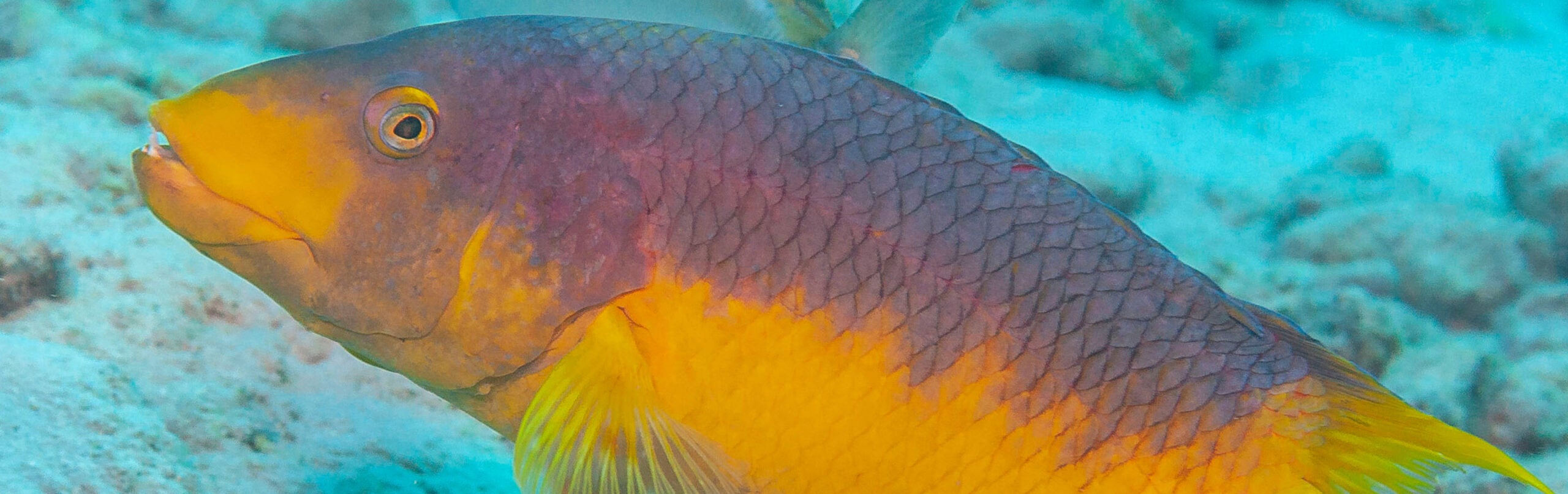This photo is a narrow, horizontally rectangular close-up of a multicolored fish swimming underwater. The fish is facing towards the left side of the frame. The background features a very light blue ocean with visible sand and some rocks, adding to the underwater ambiance. The fish's top half is a striking purple that extends down around its eye, contrasting sharply with its vibrant orange snout and belly. Its upper portion transitions towards the tail into a blend of yellow and green hues. The fish's front fin is primarily orange with transparent green tips, while the fins along its back and side showcase a gradient from orange to yellow. The fish's eye is distinguished by a black center, pink trim, and a white interior, giving the impression that it is gazing directly at the viewer. Hints of the yellow dorsal fin are also visible, making the fish's vibrant colors stand out against the serene underwater setting.